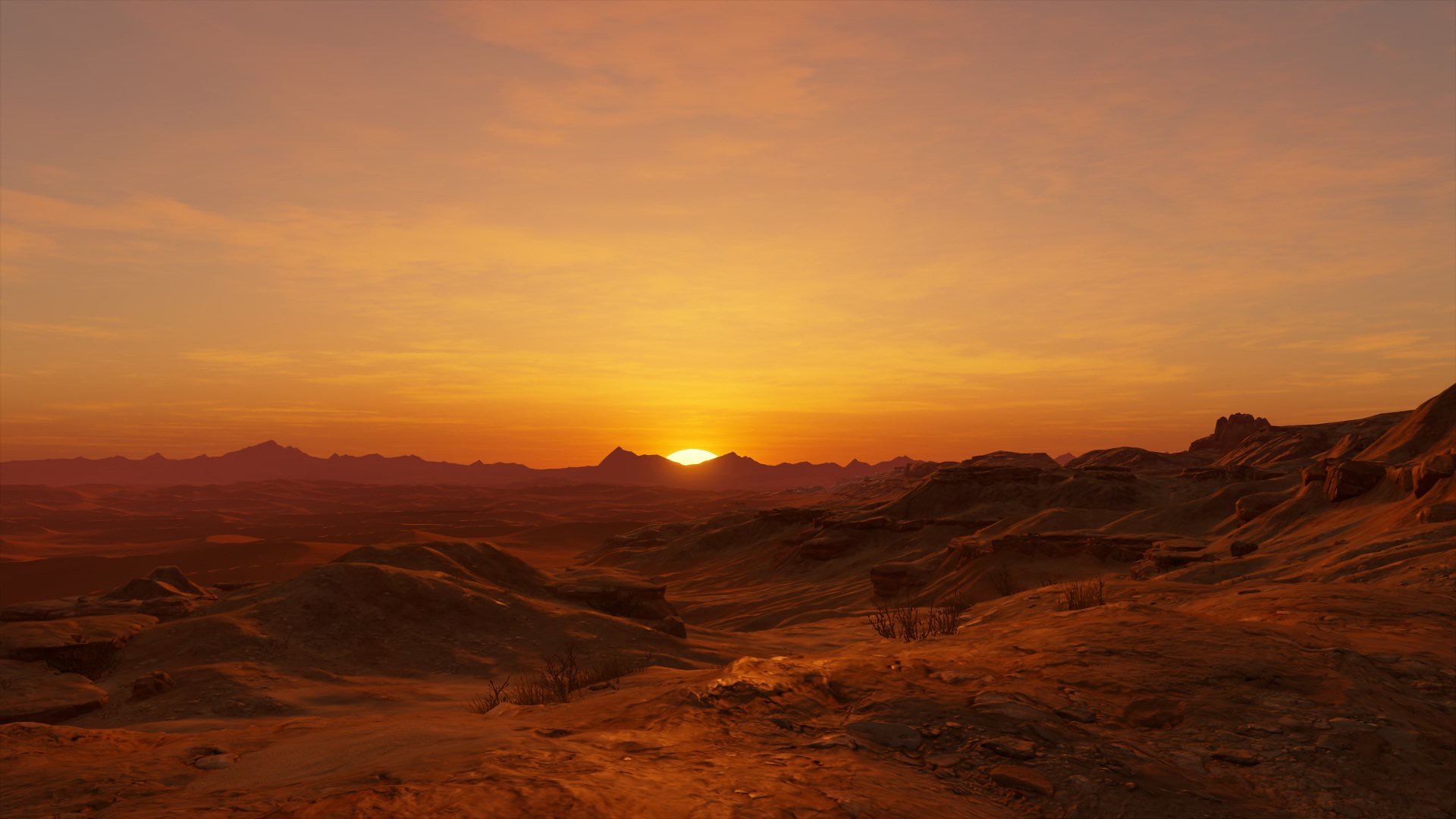A breathtaking photo captures the moment the sun, either rising or setting, gently peeks through a small gap in a distant mountain range. The terrain, characterized by its dry, dusty surface and rugged hills, stretches across the expansive desert region devoid of any signs of life. The sky is painted in vivid shades of orange and yellow, typical of dawn or dusk, with only a few scattered clouds. The low position of the sun on the horizon enhances the dramatic contrast between the illuminated sky and the stark, barren landscape, creating a surreal and tranquil scene.